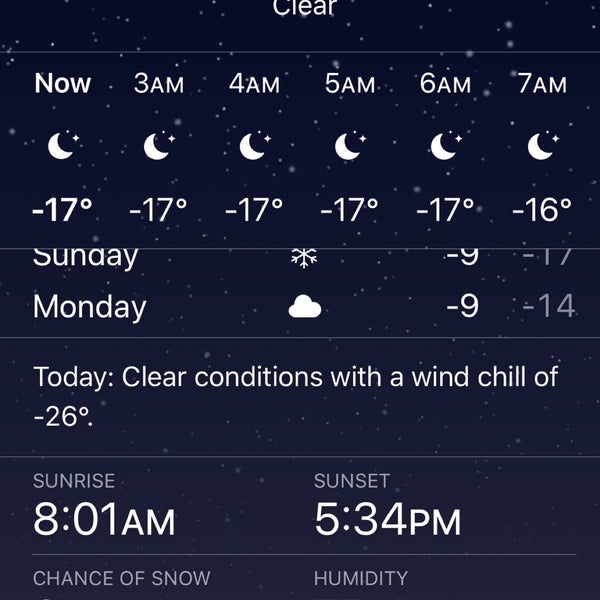The image depicts a weather app interface on a smartphone. The app features a dark, outer-space-themed background, likely indicative of the current time, which appears to be nighttime. The screen shows current weather conditions at approximately 2 a.m., with the temperature reading a frigid -17 degrees. The scale (Fahrenheit or Celsius) is unspecified. 

Hourly forecasts for 3 a.m., 4 a.m., and up to 7 a.m. display consistent temperatures of -17 degrees until about 7 a.m., where it slightly warms to -16 degrees. Below this, a five-day forecast is partially visible. The current day's forecast indicates clear conditions with an additional wind chill factor making it feel like -26 degrees, signifying extremely cold weather. Sunrise is noted to be at 8 a.m. and sunset at 5:34 p.m.

The app also displays information on the chance of snow and humidity, but this section is cut off in the image. All text and icons are white, standing out against the dark background for clear visibility.